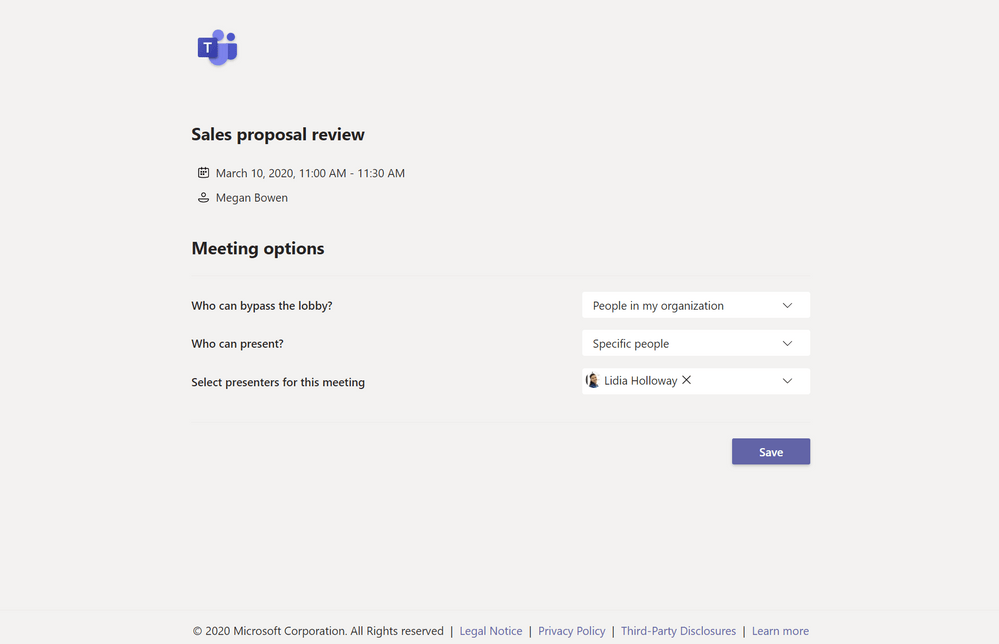Screenshot of a desktop computer displaying an online application interface with a pale white background. At the very top left corner of the screen, the Microsoft Teams logo is prominently featured; it is purple with a white capital "T" inscribed on it. Just below the logo, in bold black text, the title "Sales Proposal Review" is displayed. Further down, in smaller dark gray font, the scheduled date and time for the review is shown: "March 10, 2020, 11 a.m. to 11:30 a.m." Immediately underneath this, the name "Megan Bowen" is listed. In the lower right corner of the screen, a purple "Save" button with white text is clearly visible. The remainder of the interface, situated above this button, includes three white drop-down boxes awaiting interaction.